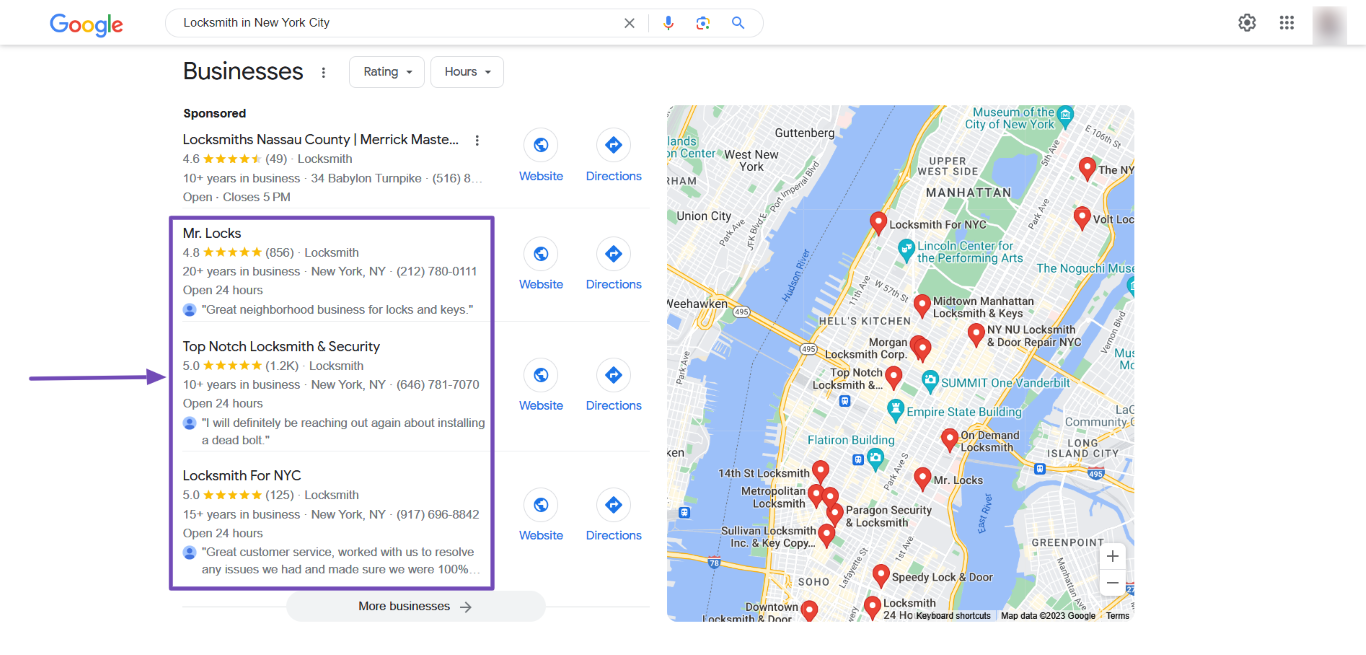The image displays the Google Maps search results page for "locksmiths in New York City." At the top, there is a thin white navigation bar bearing the Google logo in blue, red, gold, and green colors. Within the search box, the query "locksmiths in New York City" is visible, accompanied by a gray 'X' on the right for clearing the text. Alongside the search box, there are icons including a blue and red microphone for voice search, a multicolored camera for image searches, and a blue magnifying glass for initiating the search. Further to the right, a gray cogwheel represents settings, with nearby gray squares likely denoting other functionalities.

Below the search box, there's a section concentrating on black-owned businesses, featuring sorting options for rating and hours. Here, a sponsored result highlights a locksmith service in Nassau County, rated 4.6 stars based on 49 reviews, boasting over 10 years of operation. Users can access their website or get directions via blue links.

A prominent purple box spotlights three top locksmith services:
1. **Mr. Locks**: Rated 4.8 stars from over 800 reviews, with more than 20 years in business. Located in New York, New York (phone: 212-780-0111), and operates 24/7.
2. **Top-Notch Locksmiths & Security**: Carrying a perfect 5-star rating from over 1,000 reviews, with more than a decade in business. Contact: 646-761-7070.
3. **Locksmith For NYC**: Also rated 5 stars from 125 reviews, boasting 15+ years in business, with the phone number provided.

Each listing includes a brief description praising the neighborhood or emphasizing excellent customer service.

On the right portion of the image, there's a Google Maps interface showcasing the area with numerous red location pins marking locksmith services, alongside teal and white pins. The map highlights neighborhoods like Upper West Side, Manhattan, and West New York, with visible blue bodies of water delineating the geography.